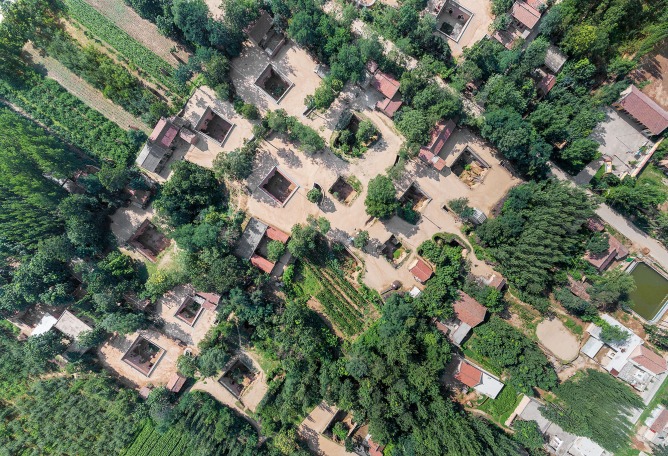This detailed aerial photograph captures the remarkable landscape of China's distinctive underground pit houses in the Loess Plateau of northern China. The image reveals a fascinating blend of architectural ingenuity and natural elements. The pit houses, appearing as square open pits, form hidden courtyards with rooms expanding laterally, seamlessly integrated into the terrain. Above these subterranean homes, lush foliage and tall trees outline the various plots, giving the appearance of a verdant tapestry. The photograph shows rows of cultivated fields and abundant greenery, including meticulously arranged garden plots and sporadic trees that demarcate the land borders. 

In the midst of these agricultural expanses, some small buildings with red roofs can be seen, possibly farmhouses or barns, along with sheds but no visible inhabitants. A central road bisects the landscape, providing a path through the verdant plots and courtyards. The area also features a pond, vital for irrigation amidst the greenery. Overall, the aerial view merges elements of rural life, agriculture, and remarkable earth-sheltered architecture, presenting a vivid glimpse into this unique way of living.